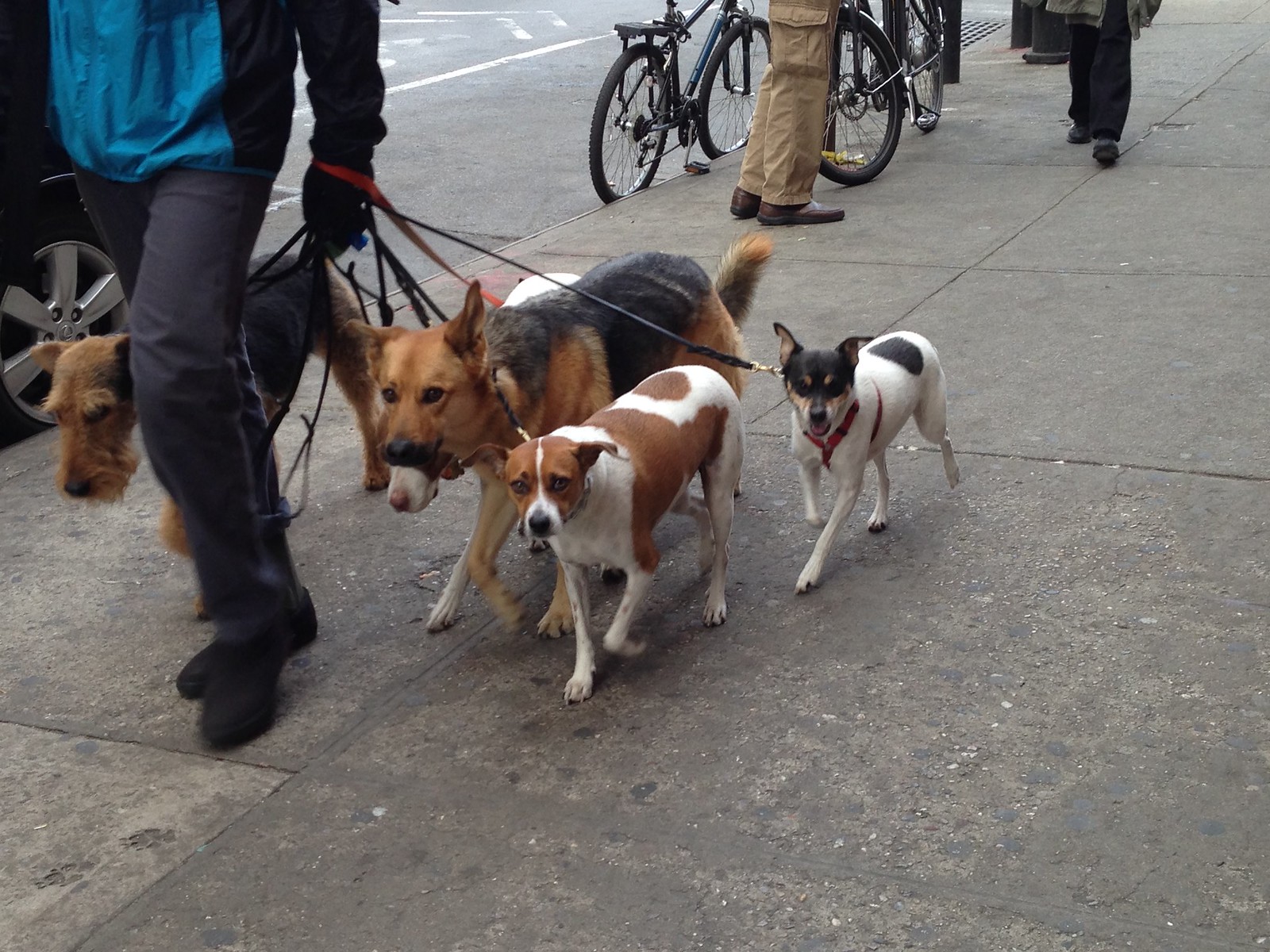In this bustling city street scene, a man wearing a black jacket over a cyan blue undershirt, gray pants, and black shoes is photographed walking five dogs on leashes. The man’s hands, covered in black gloves, tightly grip the leashes of various colors, predominantly black with one being red. The dogs, a mix of breeds, walk close together: 

- On the man's right side is a reddish-brown and black terrier, distinguished by its long snout whiskers.
- Close by is a dog with a white snout and red nose.
- A striking dog resembling a German Shepherd stands out with a black body, red face, red forearms, shoulders, and a curled black tail.
- Another dog sports a white coat with a reddish-brown triangular marking from its back extending to a predominantly brown underside, a red patch on its hips, and a white stripe running down its red face.
- The last dog is smaller, primarily white with distinctive black markings, including a large spot on its hip and a black stripe down its nose.

The city sidewalk, described as gray and somewhat worn, has a backdrop featuring additional pedestrians. One person wears tan cargo pants and dark brown shoes, and another, farther back, wears black shoes and pants with a gray open jacket. Bicycles are also visible, one being close to the man in tan cargo pants, along with a black car with silver rims parked nearby. The overall scene captures the lively interaction of humans and canines navigating the urban environment.